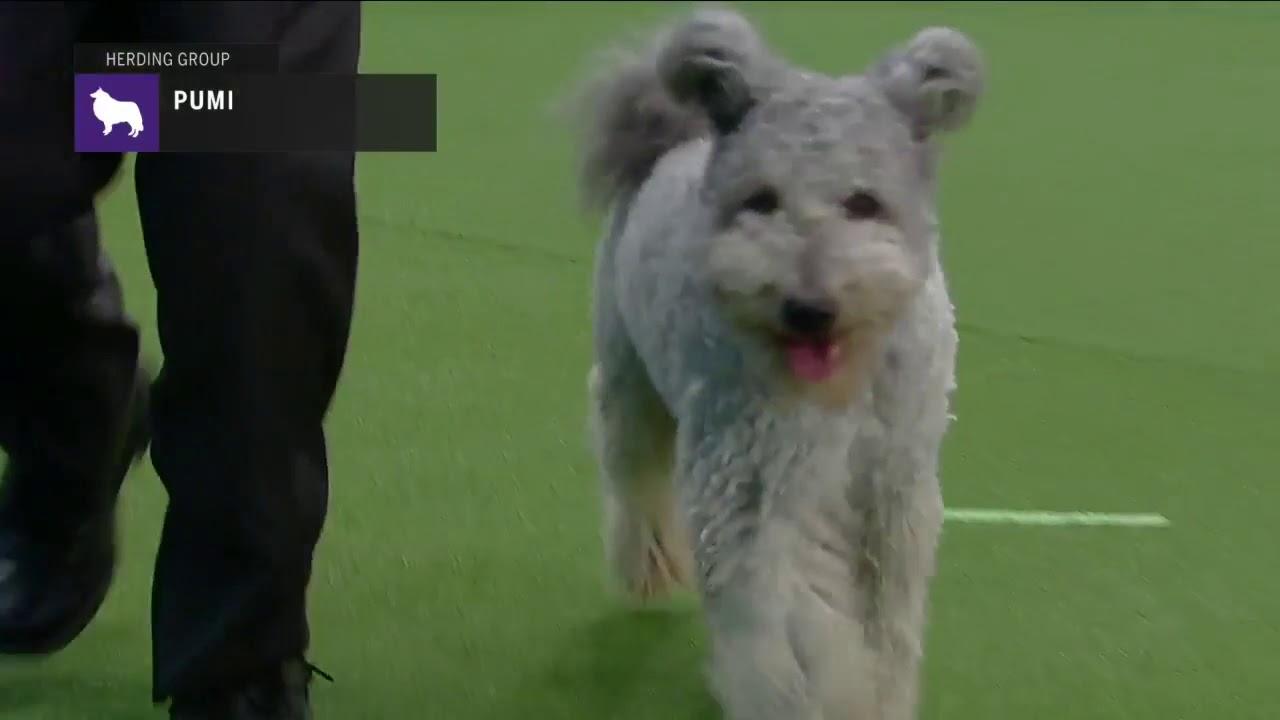This image seems to be a still shot from a dog show television program. Dominating the center is a beautiful Pumi dog with shaggy, light gray fur. The dog looks happy and content, with its tongue sticking out and its tail wagging. Its ears are particularly fluffy, adding to its endearing appearance. The background shows a person in black pants and shoes, cropped from the knees down, walking at a slow stride beside the dog. They are on a green artificial turf field, marked with a white line. In the corner of the image, there’s a simple caption that reads "Herding Group PUMI." Accompanying the text is a purple square with a white silhouette of a fancy dog, likely a logo associated with the dog show. The overall setting, which includes the dog's joyful demeanor and the clear markings on the turf, suggests a formal event where the dog is being judged.